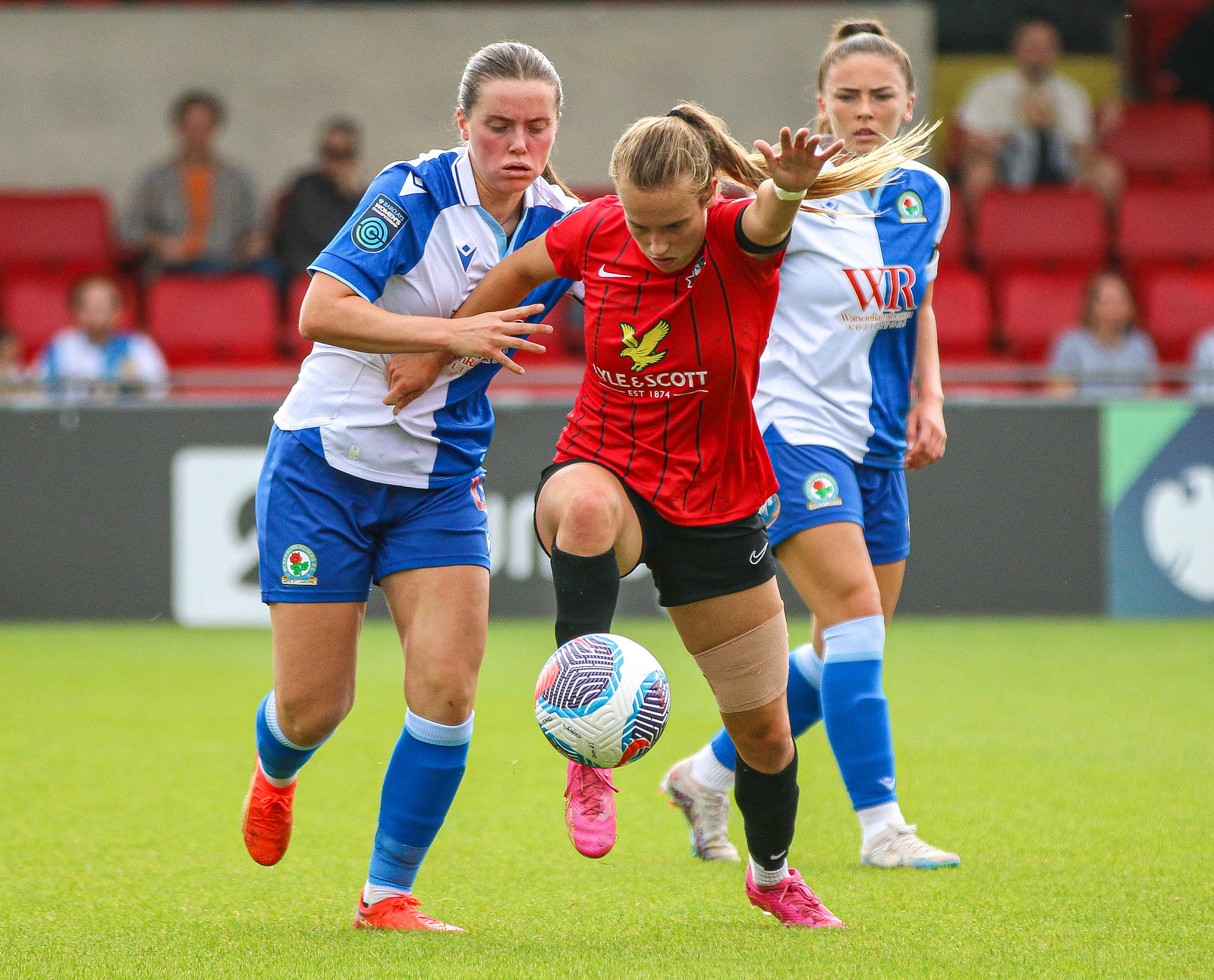The image features a dynamic scene from a women's soccer match. Center stage are three players, two from a team wearing blue and white uniforms and one from the opposing team in a red and black jersey. The blue and white uniforms consist of blue shorts, blue socks, and split-colored jerseys with "WR" and "Watson" partially visible on their tops. One player in blue has red cleats, while the other sports white cleats. Opposing them is a player in a striking red jersey with black vertical stripes, black shorts, black socks, and pink cleats. The jersey also features the text "Kyle and Scott established 1874" along with an eagle emblem. This player in red is in possession of a multicolored soccer ball (white, black, and red), while the two players in blue and white attempt to challenge her for control. The background reveals sparsely populated stands, some spectators, and an indistinct advertisement on the boards. The overall scene captures the intense action and competition in the match.